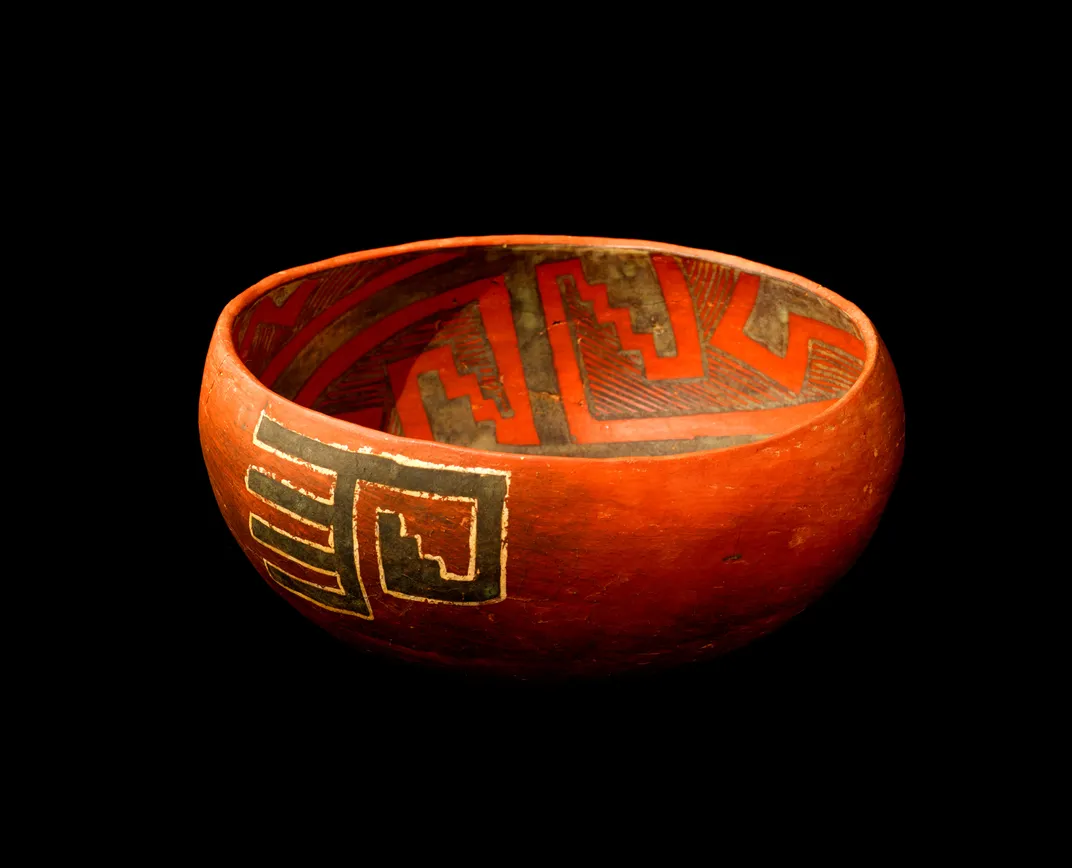The image is a rectangular photograph, about six inches wide and four inches high, with a completely black, slightly reflective background. At the center of the image is a hand-carved, round wooden bowl, possibly from a Native American or South American tribe, distinguished by its uneven texture indicating it was not machine-made. The bowl's exterior is a polished, reddish-brown hue, adorned with intricate black designs. The left side features a horizontal black bar outlined in white, with additional bars radiating from its center and extending outward in various directions, forming a geometric pattern that includes a small staircase-like figure. The inside of the bowl displays equally detailed craftsmanship, with linear designs in red and gray colors, including black diagonal stripes and staircase patterns outlined in red. The top opening of the bowl is roughly three inches wide, with the bowl standing about an inch high and its base slightly wider than the opening. Overall, the bowl and its intricate designs are centrally placed against the stark black backdrop, emphasizing its historical and artistic essence.